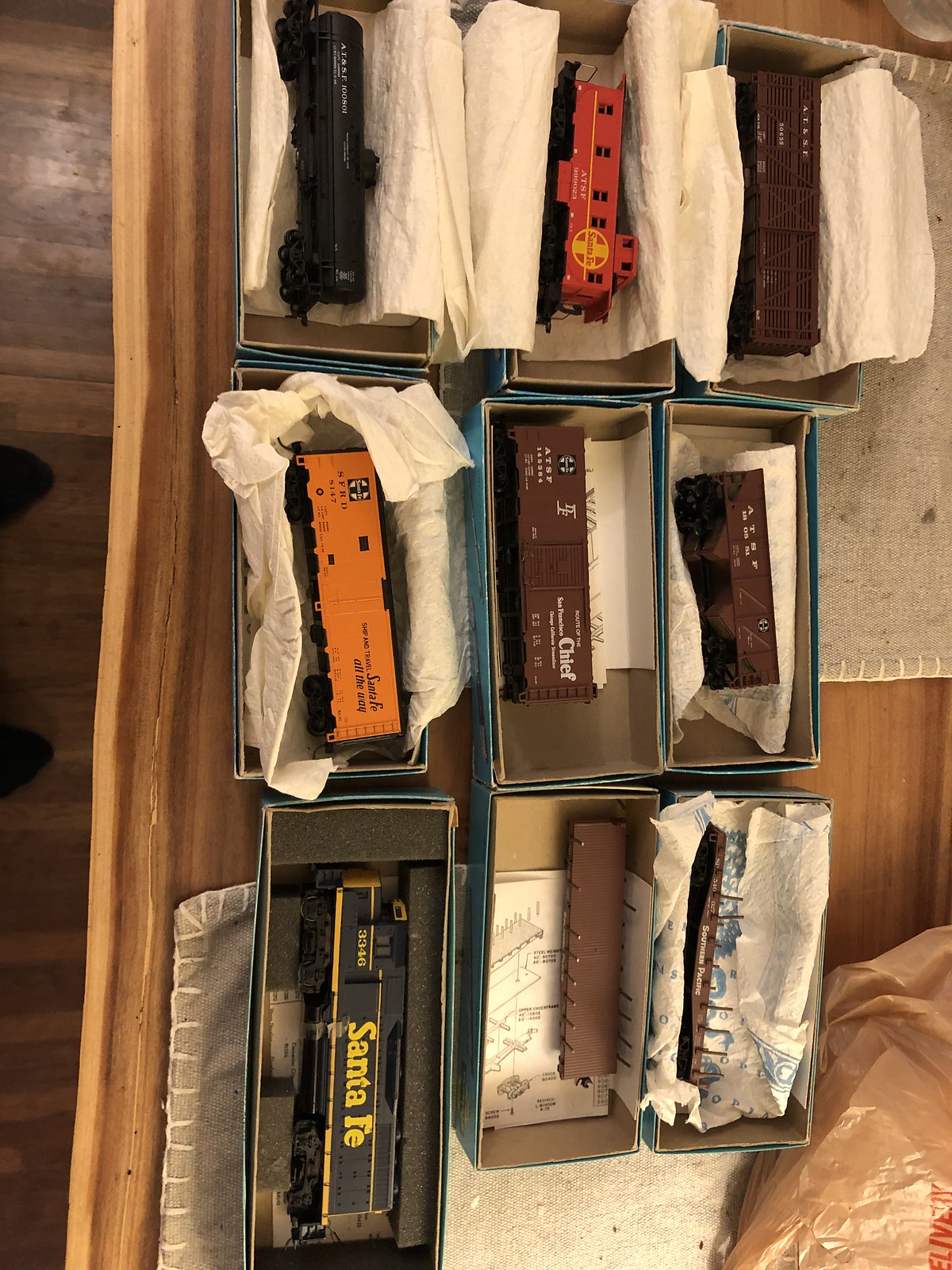This digital photograph captures an indoor scene featuring nine shoebox-sized containers, neatly arranged on a light-stained wooden table. Each box holds different pieces of a model train collection, carefully cushioned with tissue paper, foam, or cloth for protection.

Starting from the top row, the first box contains a black train car wrapped in white tissue paper. The second box reveals a red caboose with a yellow cross symbol and multiple windows, partially spilling out of its protective cloth. The third box houses a brown cargo car, also cushioned with a protective cloth layer.

In the second row, the first box showcases an orange train car with "Santa Fe" printed in black text, accompanied by a visible symbol. The second box holds a brown train car with no tissue paper. The third box contains a smaller, darker brown train car with some tissue padding.

The bottom row features a larger black engine train piece in the first box, with yellow lines and "Santa Fe" prominently displayed in yellow letters, cushioned in pieces of styrofoam. The second box includes a flat blue and yellow train component along with some instructions. The third box contains another train part secured in tissue paper and reminiscent of the previous brown cargo cars.

The table sits on a dark wooden floor with lighter wood accents, and the lower right corner of the image shows the hints of the photographer's feet and a plastic grocery bag.